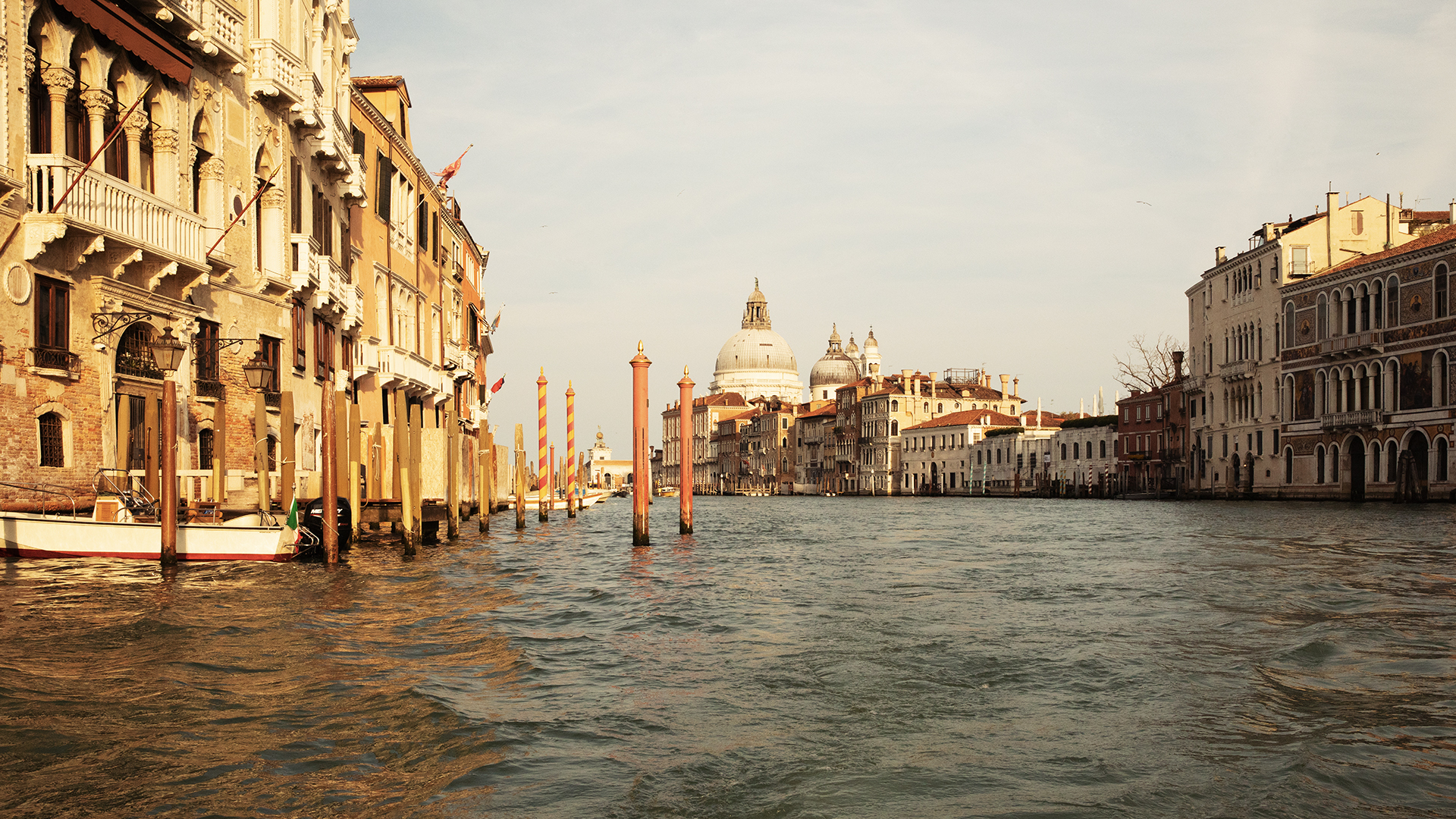This detailed, photorealistic image captures a serene waterscape scene in Venice, Italy. The canal, with its calm, subtly waved water, winds through the frame, bordered by historical European buildings that extend right up to the water's edge. The sky, shrouded in faint clouds, casts a dusty, sepia, almost warm tone, suggesting an early morning or late evening setting with the sun low in the sky.

On the left side of the image, there is an empty boat, partially tied up to red pillars emerging from the water. The tan-colored buildings on either side feature large windows, balconies, archways, and are adorned with elaborate brickwork, wrought iron street lights, and ornate decorations. In the background, domed rooftops, likely belonging to churches or significant historical structures, rise above the other buildings. The overall scene is tranquil and devoid of human activity, inviting a sense of calm and historical reverence.